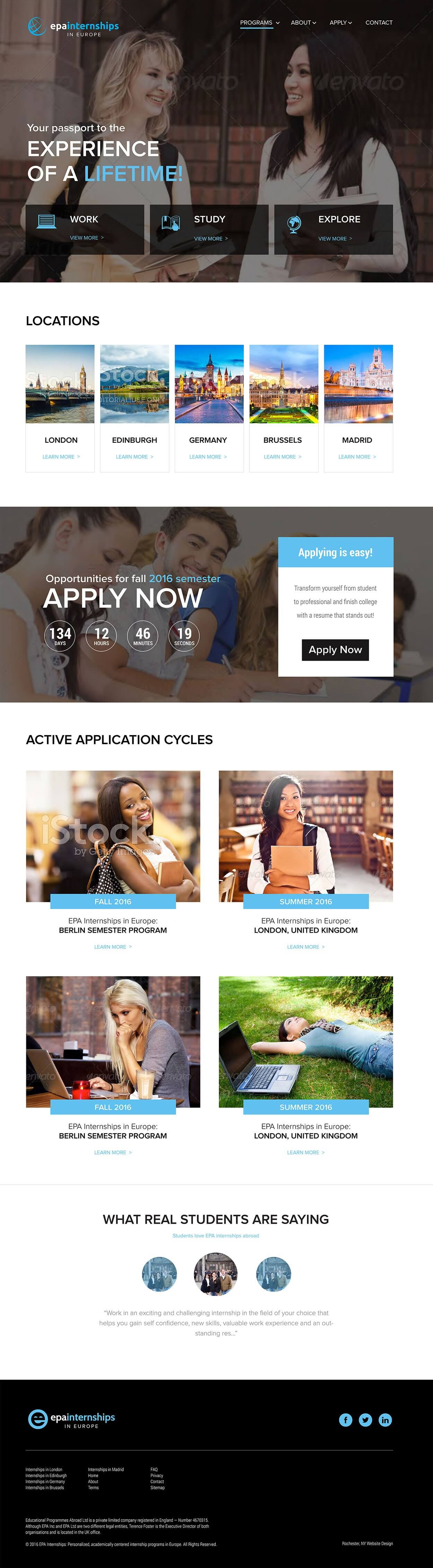The image features a visually striking advertisement for EPA internships in Europe, framed within a blue backdrop. At the upper portion of the graphic is the title "EPA Internships in Europe: Your Passport to the Experience of a Lifetime." The layout prominently displays two women wearing backpacks, one on the left and the other on the right, symbolizing the journey and exploration associated with these internships.

On the left side, there is a list detailing the opportunities available:
- **Work**: Symbolized by a laptop, with a "View More" button.
- **Study**: Represented by open books, also with a "View More" button.
- **Experience**: Encouraging exploration, with another "View More" button.

Below these categories, the image showcases various internship locations with their respective backgrounds:
- **London**: With the iconic London skyline.
- **Edinburgh**: Featuring traditional European architecture.
- **Germany**: Highlighted twice to emphasize its beauty.
- **Brussels**: Under a clear, beautiful sky.
- **Madrid**: Once again emphasized for its scenic beauty.

In the center of the image is a countdown timer, urging viewers to apply for opportunities in Fall 2016, specifying "134 days, 12 hours, 46 minutes, 19 seconds" until the application deadline. The caption encourages transforming oneself from a student to a professional, finishing college with an impressive resume. Highlighted programs include "Fall 2016," "Summer 2016," and the "Berlin Sports Program."

The image also shares testimonials from real students about the benefits of interning in Europe, like gaining self-confidence and new skills. Lastly, it depicts blue circles featuring social media icons for Facebook, Twitter, and LinkedIn, encouraging viewers to connect with EPA Internships in Europe on these platforms.